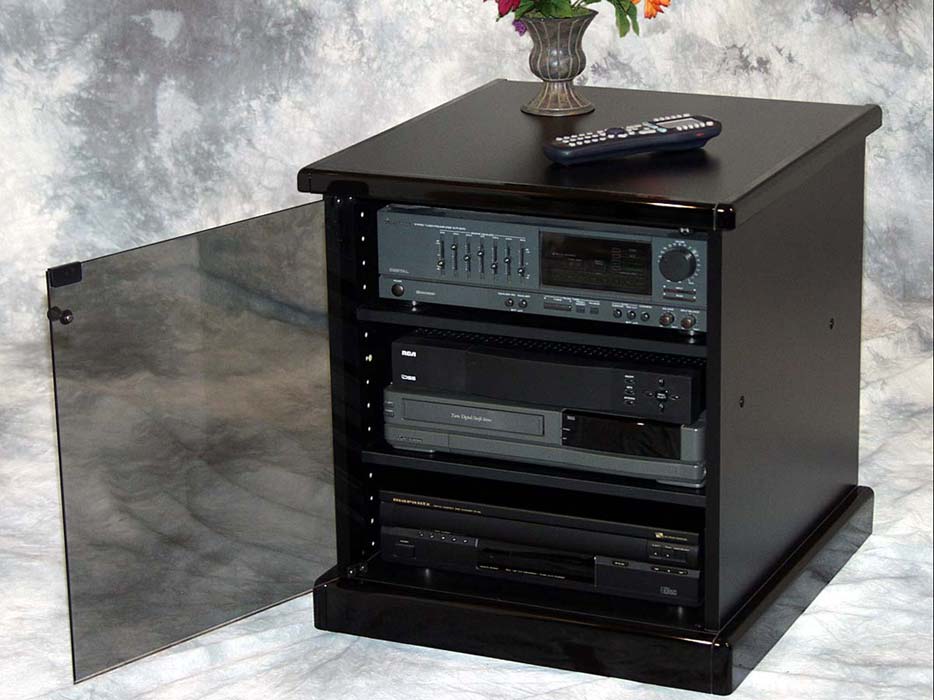This detailed color photograph captures an older-style entertainment center showcasing various nostalgic electronic devices. The main focal point is a cubic cabinet made of dark wood with a semi-transparent black glass door that opens leftward and is secured by a magnetic latch. Inside, we can see three distinct entertainment devices: a VHS player, a stereo system with adjustable treble, bass, and balance knobs, likely a cassette player, and possibly a CD or DVD player. All these components reflect a bygone era of home entertainment. Resting on top of this cabinet is a black remote control with white buttons, used to operate the three electronic devices inside. Additionally, there is a vase adorned with orange flowers, slightly draping down. The entire setup is staged against a sophisticated backdrop of white and grayscale marble that runs from floor to ceiling, accentuating the retro aesthetic. This photograph appears to be meticulously arranged, possibly for an advertisement, providing a nostalgic glimpse into past entertainment setups.